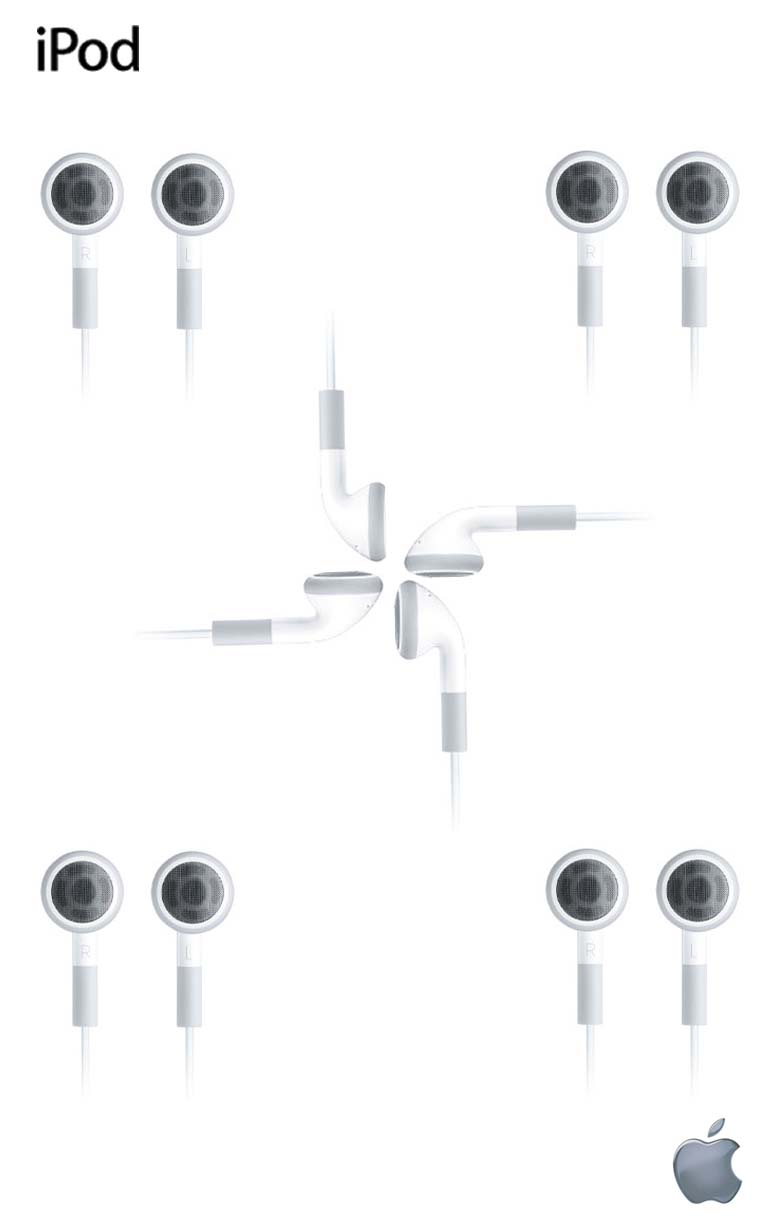This image depicts a detailed arrangement of classic Apple wired earbuds on a white background. In each of the four corners of the image, there is a pair of these old-style, white earbuds, with the earpieces facing outward towards the viewer, highlighting the L and R designations. At the center of the image, four additional earbuds are positioned on their sides, forming a cross or square shape with the cords radiating toward each edge. The mesh of the earpieces is translucent, revealing some white plastic inside. The composition creates a symmetrical and somewhat puzzled aesthetic. Notably, the bottom right corner features a small silver Apple logo, subtly anchoring the visual as a creative yet controversial nod to the brand's historic, early 2010s earbuds.